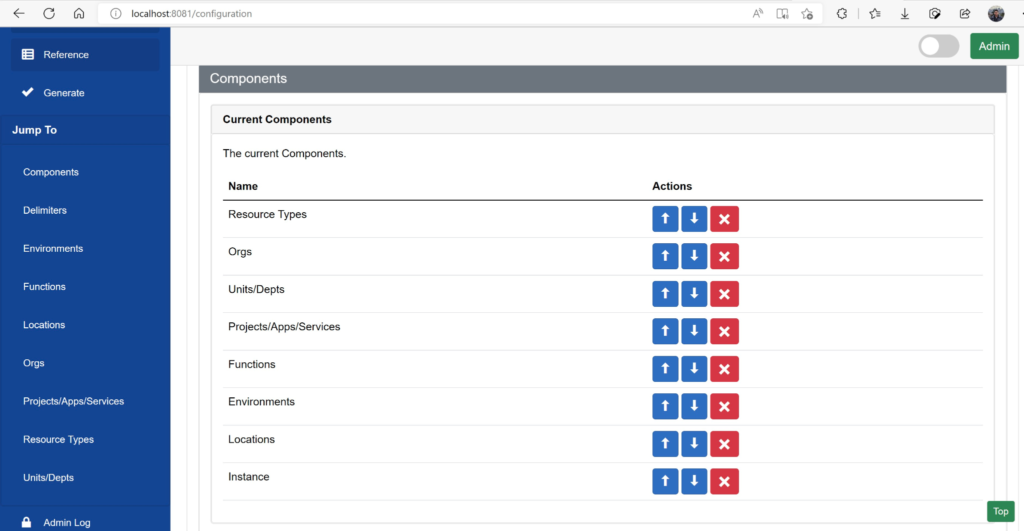The image presents a screenshot of a web page displaying a configuration interface, likely for a local development server (localhost:8081/configuration). At the top of the page, standard browser navigation elements are visible: a back button, a refresh button, a home button, and a web address bar indicating the URL. Additional icons for bookmarks, downloads, a camera, and forwarding are also present, along with a profile picture depicting a man, suggesting the user is logged in.

On the left side of the page, there is a vertical blue panel featuring navigation options written in white text. This panel includes links to various sections such as "Reference Generate," "Jump to Components," "Environments," "Functions," "Locations," "Orgs," "Project/App/Services," "Resource Types," "Units," and "Departments." A lock icon at the bottom indicates restricted access to admin logs.

The main content area on the right side of the page, set against a white background, lists "Components" and "Current Components" with corresponding "Name" fields. Users can interact with blue buttons for uploads and downloads, and red buttons with X's for deletion. An "Admin" button in green is prominently displayed at the top, indicating options for administrative actions.